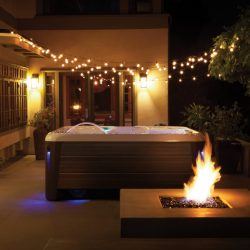The image is a color photograph taken outdoors at night, primarily black around the top and edges, capturing a cozy outdoor patio scene. Dominating the foreground is a rectangular table with a central, blazing white and yellow flame, suggestive of an outdoor fireplace pit, on the bottom right. The surface of the table appears white, potentially covered with ice, and a little bluish-green drink is visible protruding from the left side. Behind the table sits a jacuzzi tub with a dark wood exterior and a white rim; under its left corner, a soft blue glow emanates. In the background stands a white stucco building with two hanging, bright white and yellow exterior lights flanking sliding glass doors. Additional ambiance is provided by several strands of small, hanging lights strung across the area, softly illuminating the patio. The photograph is square in format and adheres to a style of photographic representational realism.